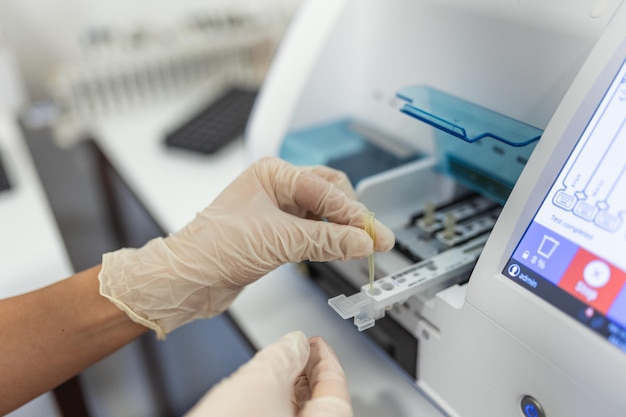The image captures a detailed scene in a laboratory where an individual is meticulously handling liquid samples. The person, wearing beige latex gloves, is in the process of pipetting a liquid into a small slot on a sophisticated analysis machine. This machine, reminiscent of an ATM in appearance, is designed to house multiple rows of miniature pipettes in a holder with a translucent blue lid that slides down to secure the samples. The lab worker’s left hand is prominently visible, while only the fingers of their right hand can be seen. To the right of the machine, a screen displays several operational buttons, including a stop button, a trash button, and a profile showing an admin interface. Additionally, on a blurred desk adjacent to the setup, a calculator is faintly visible. The image underscores a precise and methodical approach to liquid sampling within this scientific environment.